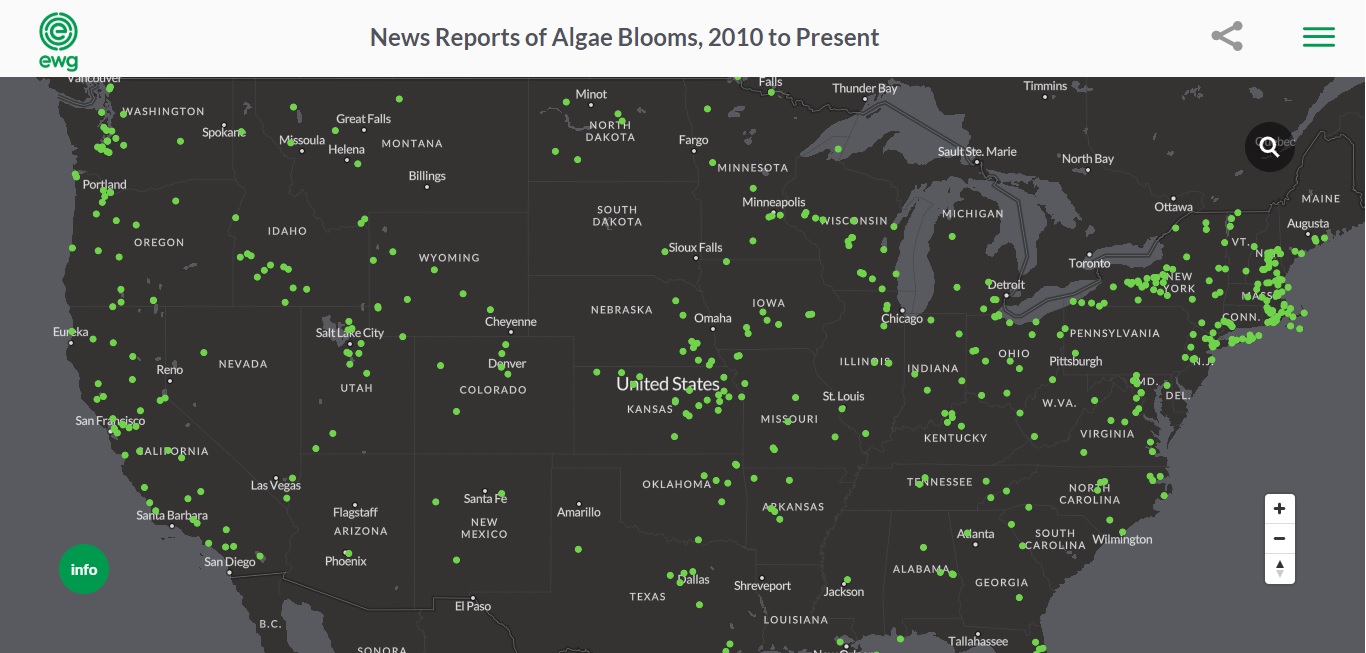**Descriptive Caption:**

This image is a detailed screenshot of a web page featuring a map of the United States. The map is primarily black, with the names of the states and select towns written in white letters, typically highlighting one town per state. Scattered across the map are numerous green dots, which represent various pieces of information. To the left of the map, there is a small green circle labeled "info." The background of the entire web page is a dark gray color.

On the right side of the map, there are plus (+) and minus (-) buttons for zooming in and out. In the top right corner, a search icon is visible. Above the map, a white bar spans the width of the page. Within this bar, on the left-hand side, there is a green circle containing the letter "E," with the text "EWG" written underneath in green.

The title positioned above the map reads "News Reports of Algae Blooms, 2010 to Present." Adjacent to this title, on the right, is a share icon. Near the upper right corner of the screen, there are three green horizontal bars that can be clicked on for additional information.